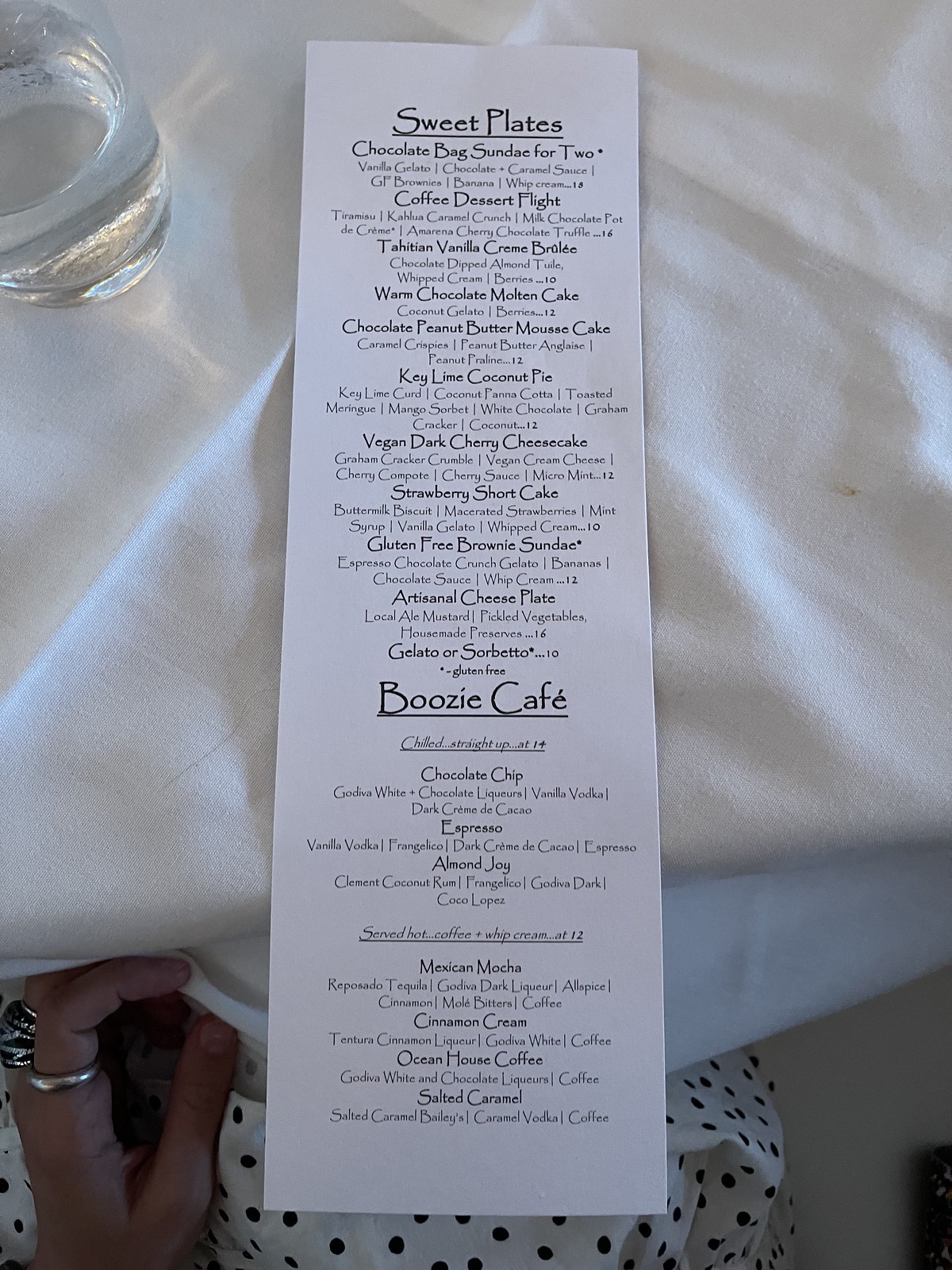This image features a white receipt, which is notably long, lying on a surface that resembles a white tablecloth. The top of the receipt prominently reads "Sweet Plates," followed by a detailed list of various dessert items. Beneath this section is another labeled "Boozy Cafe," which also contains a list of items, though they are somewhat difficult to read. Adjacent to the receipt, there is a white garment adorned with black polka dots. In the lower left-hand corner of the image, a woman's hand is visible, adorned with a large ring on her index finger. In the top left-hand corner, there is a glass of what appears to be water. The background is mostly white and blends with the tablecloth, creating a clean, minimalistic setting.